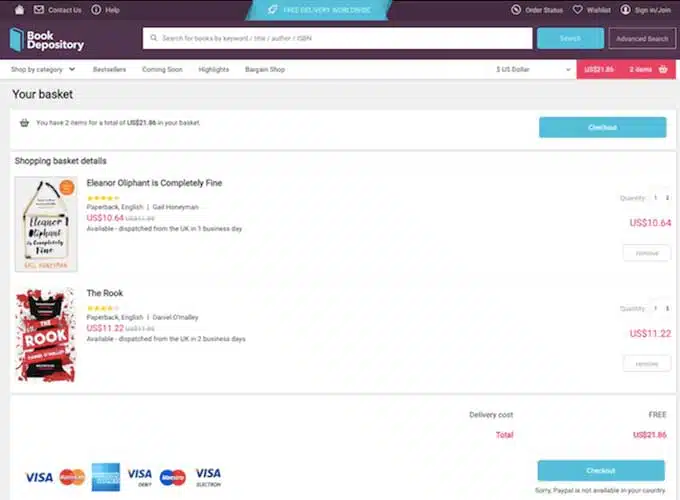The image depicts a computer screen showing an online library's shopping interface, specifically from the Book Depository website. At the very top, there's a dark brown navigation bar with options such as "Contact Us" and "Help". Below it, in a blue box, the site advertises, "Free Delivery Worldwide".

Further down, another navigation bar includes options: "Order Status", "Wish List", and "Sign In/Join". Underneath, a thicker bar reads "Book Depository" and features a search bar along with an "Advanced Search" option on the right.

Immediately below, a white bar displays categories such as "Shop by Category", "Best Sellers", "Coming Soon", "Highlights", and "Bargain Shop". The right side of this bar indicates the currency as "U.S. Dollar" and shows the shopping cart information.

The cart summary reveals that there are two items in the basket totaling $21.86. The items listed in the shopping basket include:

1. "Eleanor Oliphant is Completely Fine" by Gail Honeyman, priced at $10.64, noted as a paperback in English, with availability for dispatch from the UK within one business day. A small image of the book is also displayed on the left.
2. "The Rook" by Darcy O'Malley, priced at $11.22, also a paperback in English, with the same dispatch conditions from the UK.

The total cost of these items is $21.86, with free delivery. The accepted payment methods are Visa, MasterCard, American Express, Visa Debit, and Visa Electron. However, there is a note that PayPal is not available for use in the current country of the user.